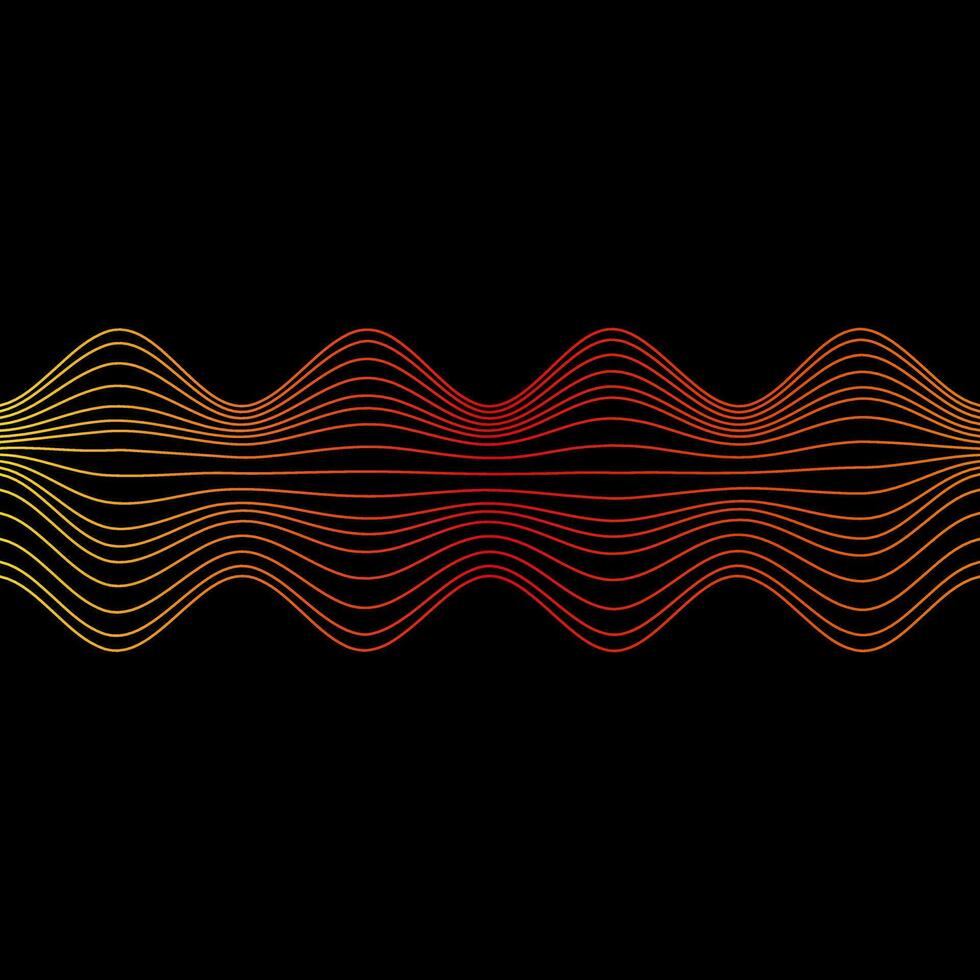The digital artwork features a flat, unchanging black background across which runs a series of twelve multicolored lines. These lines flow horizontally, much like the depiction of sound waves or radio signals. The lines exhibit a mesmerizing wave pattern: starting relatively straight in the center and curving more pronouncedly toward the top and bottom edges, creating a rhythmic visual oscillation. They boast a vibrant color gradient, transitioning from yellow at the edges to orange, culminating in a deep red in the middle, and then reversing the gradient back to yellow. The lines also emit a subtle glow—though primarily enclosed by a black border—that slightly alters the shades of the black background, adding depth and visual intrigue. This neon gradient and dynamic wave pattern make the artwork striking and eye-catching.